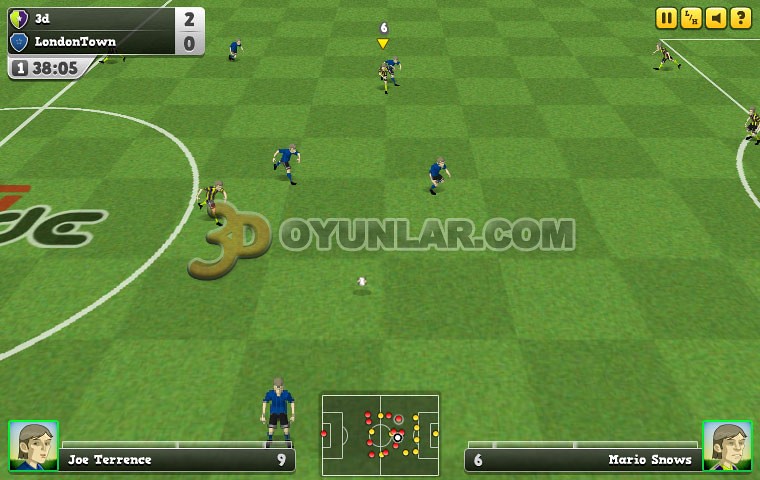The image depicts a still from a video soccer/football game, focusing on a segment of the pitch angled slightly to the right. The pitch is presented in a checkerboard pattern featuring alternating medium and dark green squares, reminiscent of a textured velvet. In the upper left corner, the top section of the partially visible center line appears as a slanted white line. The upper right corner reveals the edge of the goalkeeper's box and a portion of the white semicircle surrounding it, although the goal itself is not visible.

The scene centers around a few players animated on the field. The home team, wearing blue shirts and black shorts, consists of five visible players. One player is standing idle in the lower center of the image, facing the stands. The opposing team, clothed in black and yellow vertically striped tops with black shorts, includes three players spread across the pitch; two near the top of the goalkeeper's box. Players Joe Terrence (number 9) and Mario Snows (number 6) are specifically indicated as controlled characters. Their names, accompanied by shoulder-up avatars, appear in the lower left and right corners, respectively.

Overlaid in the image's center is light brown 3D text with the gray, white-outlined URL ‘Oyunlar.com’ below it. Right beneath this text, the soccer ball is clearly visible. At the top, a scoreboard indicates the home team 3D leads London Town by 2-0 in the first half, showing a game time of 38:05, and includes logos for each team—with 3D’s in purple and yellow and London Town’s in blue. The image also features a mini-map in the bottom center showing player positions with red and yellow dots, and icons for pause, sound, and a question mark in the upper right corner.

Overall, this snapshot provides a detailed, comprehensive view of a dynamic moment in the video soccer game's immersive stadium setting.